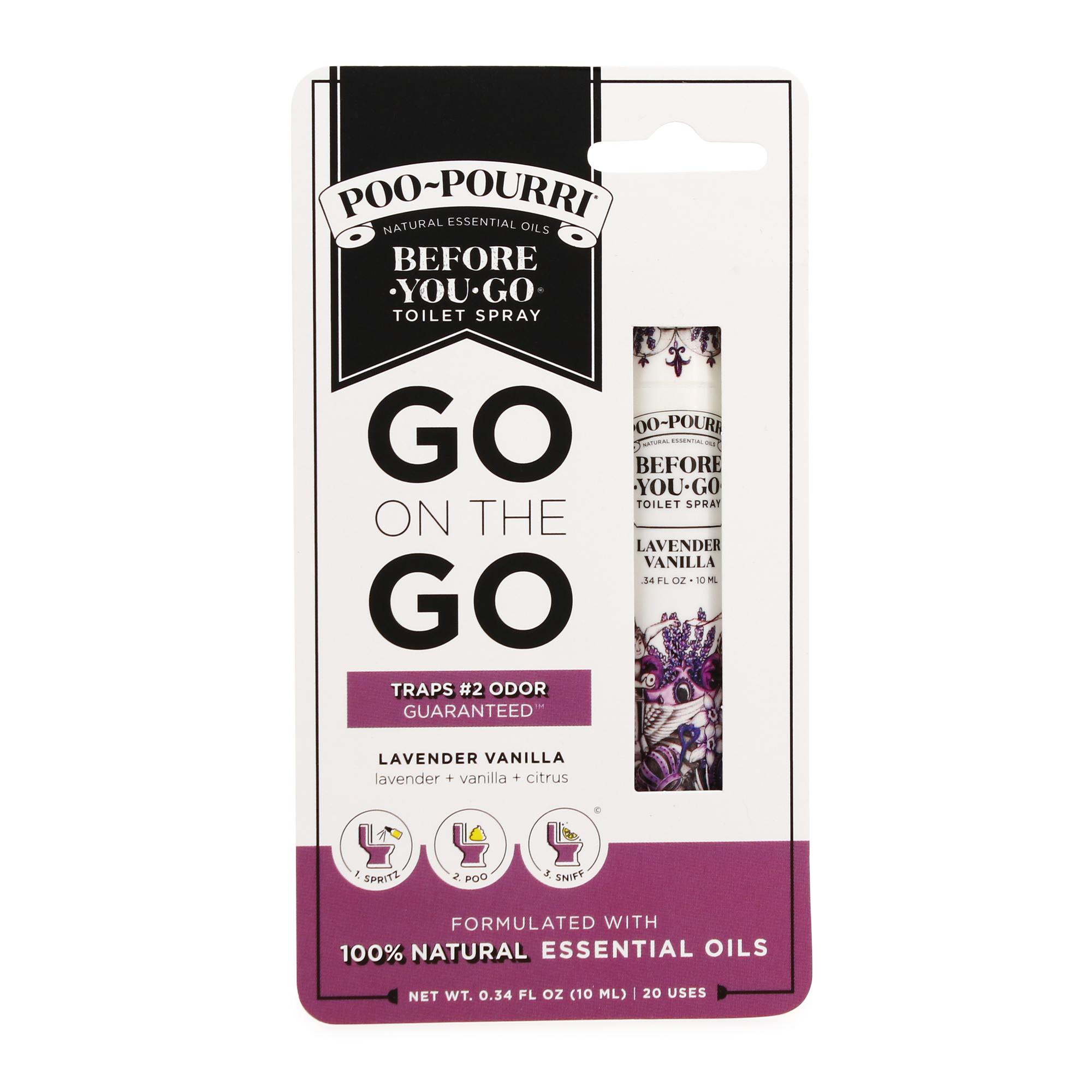The image advertises a product called Poo-Pourri, specifically a toilet spray designed to trap bathroom odors using natural essential oils. The packaging prominently features the name "Poo-Pourri" along with the tagline "Before You Go Toilet Spray." The product variant showcased is "Lavender Vanilla," which also includes hints of citrus, as indicated beneath the product name. 

On the right side of the package, there is a small window displaying the cylindrical spray bottle, which is labeled "Before You Go Toilet Spray, Lavender Vanilla." The packaging is mainly white with black and purple accents; the top two-thirds are white, and the bottom portion transitions to purple. 

The left side of the package explains the product’s function, stating it can be used "on the go" and guarantees to trap number two odors. Below this, a black banner reads "Lavender Vanilla, Lavender + Vanilla + Citrus," and there are illustrations with instructions: "Spritz" into the toilet bowl, "Poo" (indicated with an icon of a person using the toilet), and "Sniff." 

At the very bottom, it is noted that the spray is "Formulated with 100% Natural Essential Oils," and the net weight is specified as 0.34 ounces (10 milliliters), sufficient for about 20 uses.